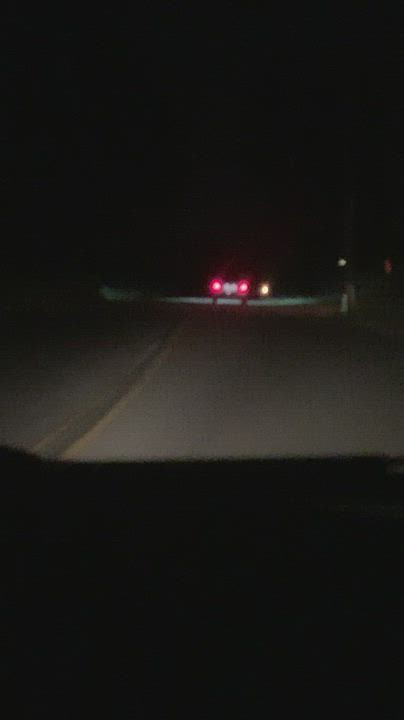In this dark photograph taken from inside a car, the roadway ahead is visible, revealing a narrow, one-lane road supporting traffic in both directions. The only illumination comes from the headlights of vehicles, which cast a stark contrast against the night. Up ahead, a car is seen with its brake lights glowing red, piercing through the darkness. The silhouette of the dashboard frames the lower part of the image, adding an intimate perspective from within the car.